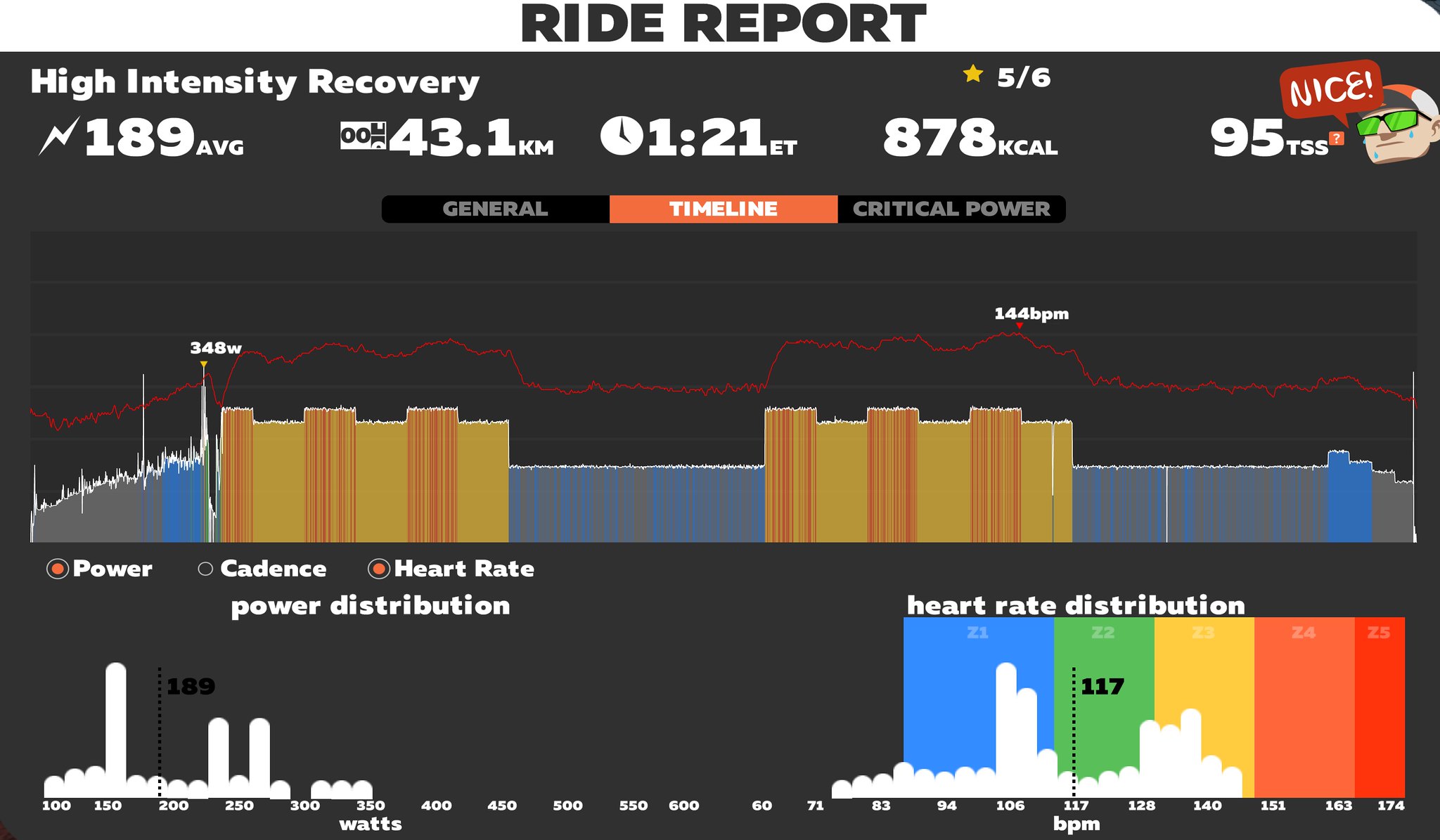The image is an infographic titled "Ride Report" with a dark gray background. At the top, it displays the text "High Intensity Recovery" in white, accompanied by a lightning logo and several key statistics: "189 average," "43.1 kilometers," "1.21 ET," "878 Kcal," and "95 TSS." In the upper right corner, there's a small graphic of a face with green glasses and a sweat or tears icon, wearing a white hat with a red stripe, saying "Nice."

The infographic appears to track various performance metrics related to a ride or workout. The metrics include power (measured in watts), cadence, heart rate (BPM), and power distribution. The main section features a large graph visually depicting these statistics, and the bottom of the image contains additional graphs for power distribution and heart rate distribution. These elements collectively provide a detailed summary of the ride's intensity and effort.